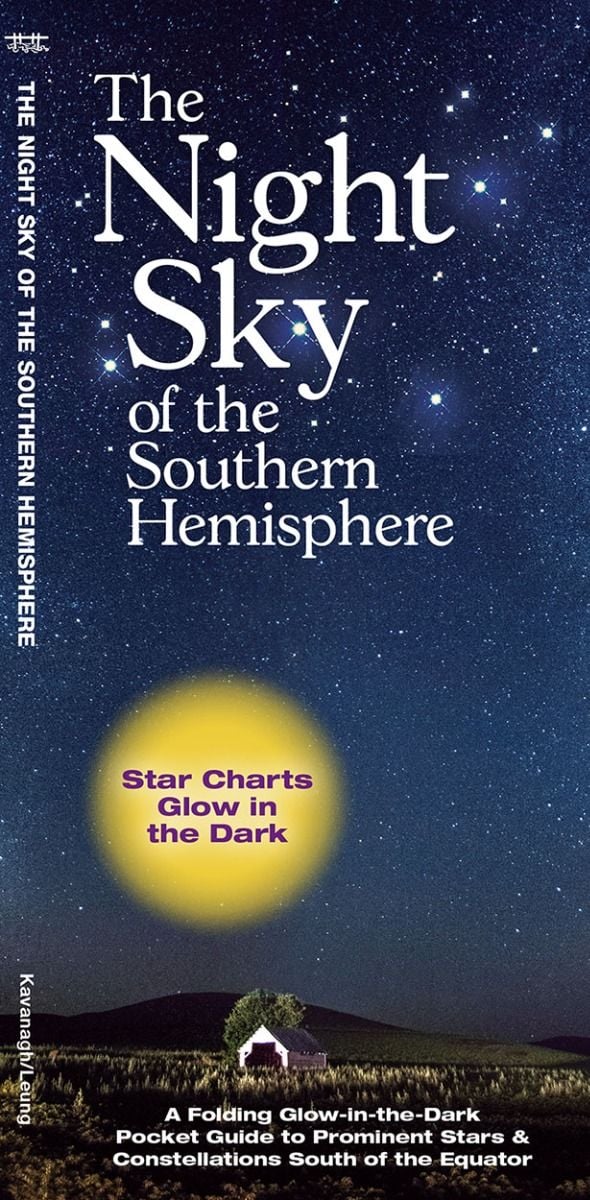This image features the cover of a folding glow-in-the-dark pocket guide titled "The Night Sky of the Southern Hemisphere." The title is prominently displayed at the top in large white letters. The background of the cover showcases a stunning dark blue night sky filled with numerous white speckled stars and the Milky Way, with a bright yellow moon icon that declares, "Star Charts Glow in the Dark." Below the celestial display, the scene transitions into a serene landscape with a rolling prairie hill, a small white farmhouse with a black roof, and a single tree. Towards the bottom, the text reads, "A folding glow-in-the-dark pocket guide to prominent stars and constellations south of the equator." The guide is authored by Cavanaugh Leung. This visually captivating cover integrates the vast beauty of the Southern Hemisphere's night sky with a tranquil rural setting, making it both informative and visually appealing.